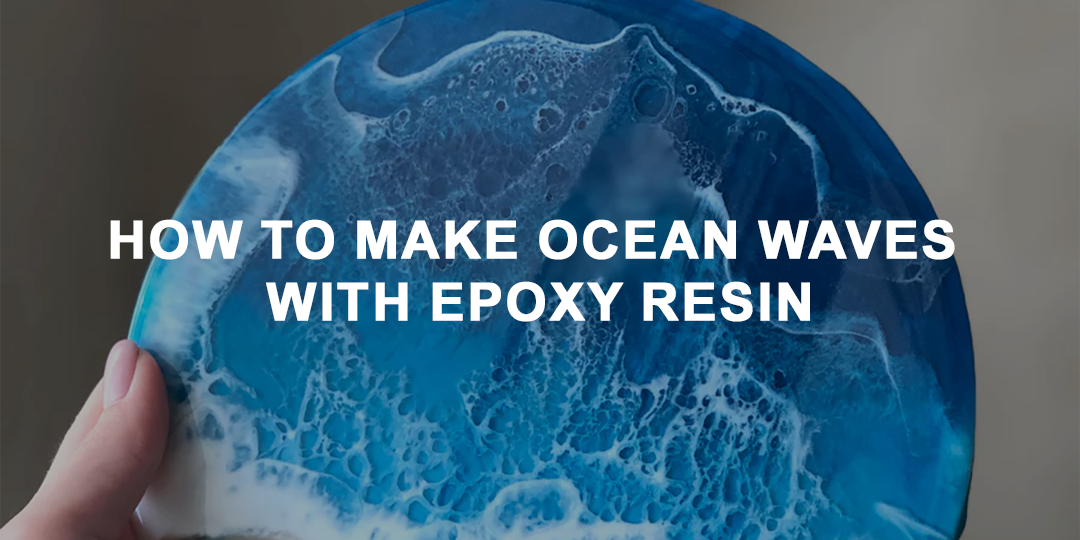The rectangular, horizontal image is a visually captivating tutorial thumbnail. Central to the image is a circular, blue object, resembling a plate or a globe, intricately designed to mimic ocean waves using epoxy resin. A woman's hand, adorned with pink nail polish, is prominently featured on the lower left, holding the object with her thumb and forefinger. The blue surface of the object showcases a striking 3D wave effect, transitioning from dark blue at the top to a lighter blue at the bottom, with realistic white accents that emulate the frothy crests of waves. The background of the image is a gradient of light and dark browns, complementing the gray backdrop that contrasts with the vivid blue of the circular object. Dominating the top of the image, large, bold white letters announce, "How to Make Ocean Waves with Epoxy Resin," immediately capturing the viewer's attention and hinting at the beginning of a detailed tutorial.